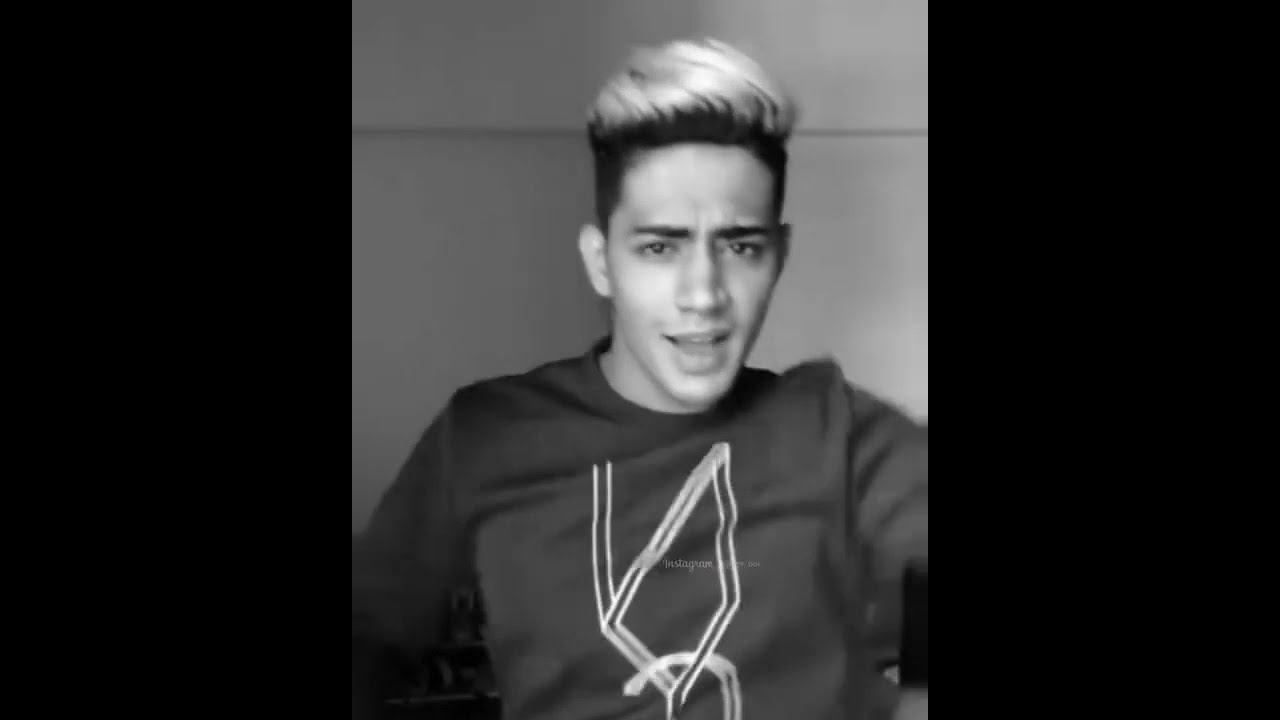The black-and-white photograph features a young man, possibly of Latino descent, leaning back in a chair and captured from the mid-waist up. The image is rectangular with black borders on both the right and left sides, making the central picture stand out. The young man has distinctive two-toned hair: the sides are dark, while the top is bleached blonde and styled into a bouffant that swirls to the right, resembling an ice cream cone. He appears to be in the middle of talking or perhaps exclaiming something cheerful, with his mouth open and a faint smile. He wears a lightweight, long-sleeved shirt adorned with an abstract, geometric design that vaguely resembles a letter U with a line through it. The image is slightly out of focus, and behind him is what appears to be a wall with large siding. The word "Instagram" is faintly visible across his chest, indicating the platform where the photo might have been shared.